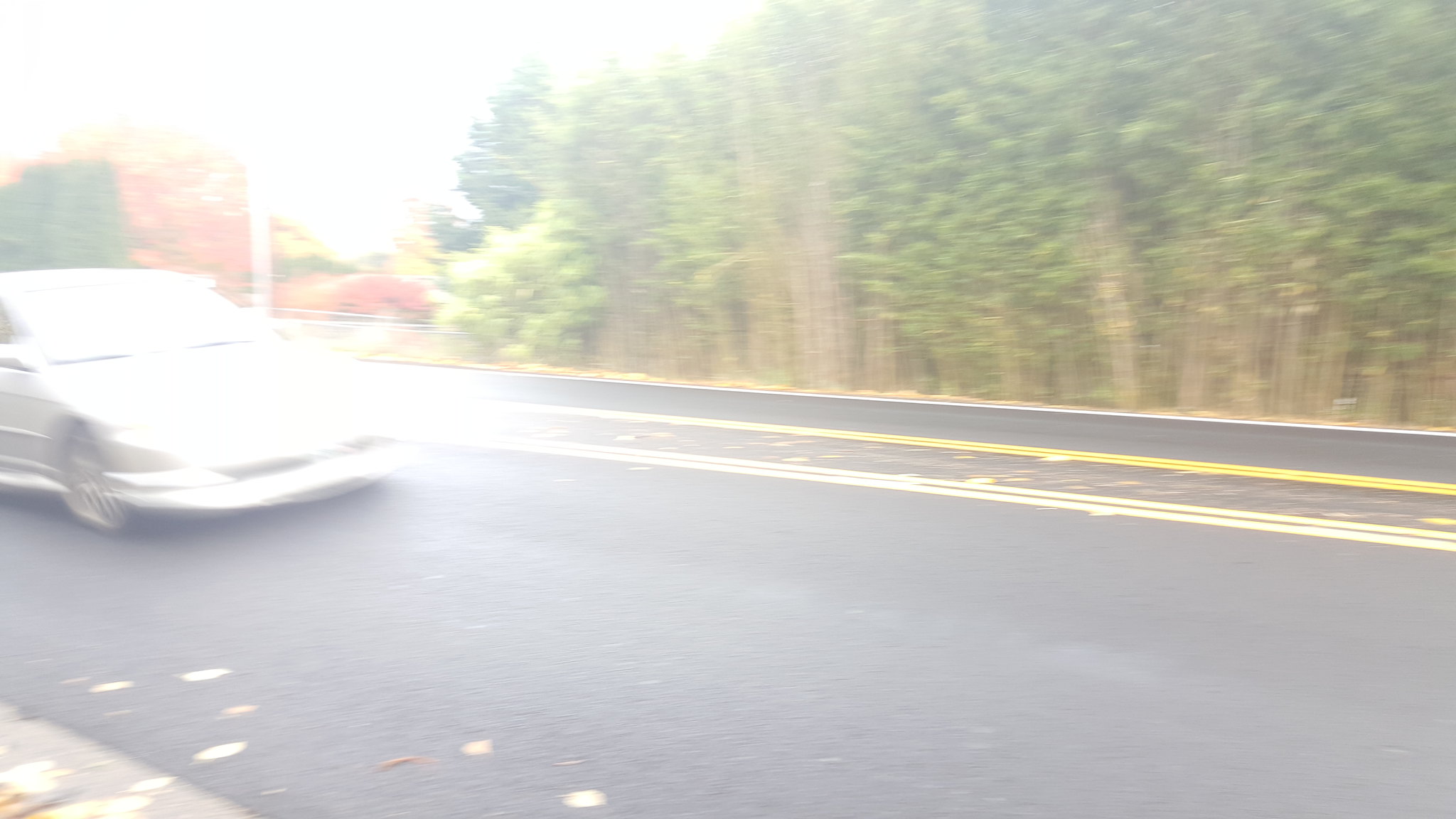A daytime color photograph captures a slightly blurry scene, washed out by intense sunlight, with noticeable lens flare. The image features a two-lane highway with a wide median that includes a double white line and a double yellow line. The road, with black pavement, has some white dots in the lower left corner, likely due to the photo's exposure. A light-colored, possibly silver car is positioned on the extreme left, heading towards the right side of the frame.

In the background, the scene is lined with a diverse array of trees. Deciduous trees in various shades of green, ranging from light to dark, mix with some bearing orange and yellow leaves. These trees have thin trunks, with hints of brown visible. The upper left-hand corner is dominated by a very bright and almost completely obscured sky, which spills light across the scene, further contributing to the blurred effect.